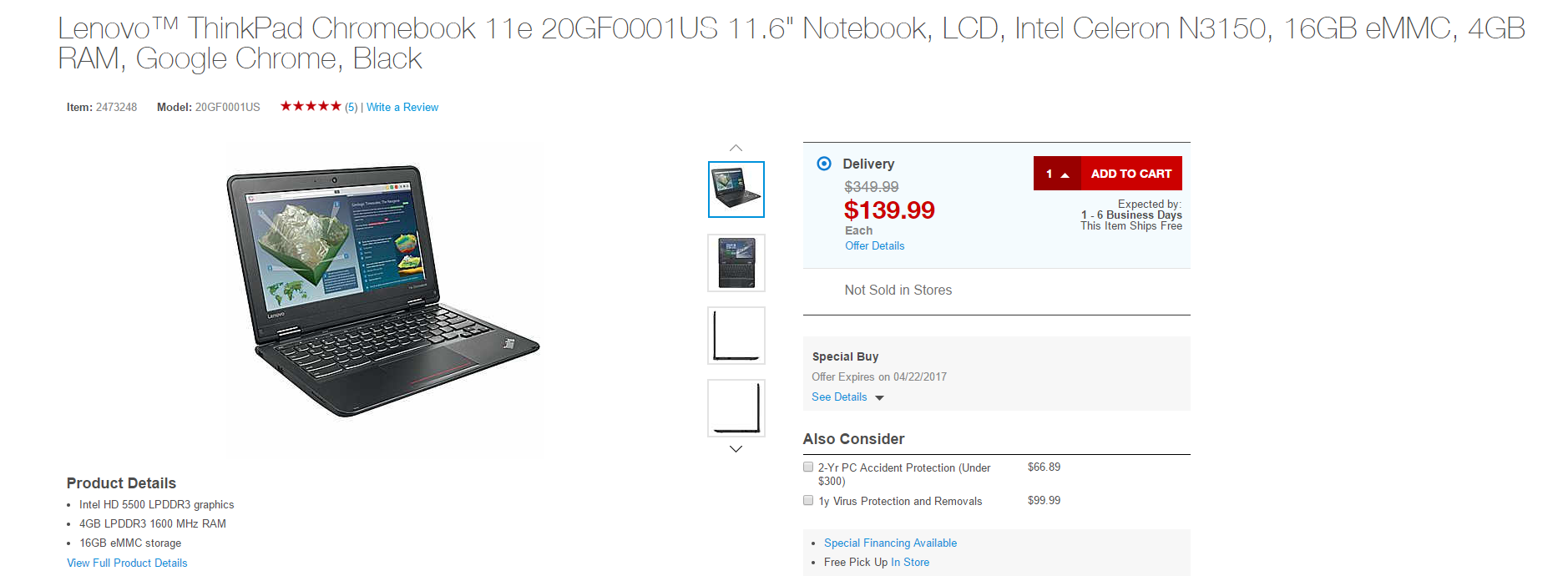The image is approximately two and a half times wider than it is tall, featuring a white background that obscures its edges. At the very top, there's thin gray text reading: "Lenovo ThinkPad Chromebook 11E20GF0001US, 11.6-inch notebook, LCD, Intel Celeron N3150, 16GB eMMC, 4GB RAM, Google Chrome, black."

Below this text is a review section displaying five stars, though the descriptive text is not entirely clear. Three mentions of this rating can be seen on the left-hand side.

The central part of the image showcases a black Lenovo ThinkPad Chromebook angled slightly, resembling a 4:35 clock position. The laptop's screen displays a blue background with a 3D model on the left side. 

To the right of the laptop, there is a purchasing section. At the top, it indicates delivery options. The original price of $349.99 is crossed out and replaced by the current price of $139.99, highlighted in red. In the upper right corner of this section is a prominent red "Add to Cart" button.

Further down on the left side of the image, there's a note stating "Not Sold in Stores," followed by smaller, unreadable text. The bottom of the right-hand side contains a section labeled "Also Consider," suggesting add-on items with accompanying visuals.